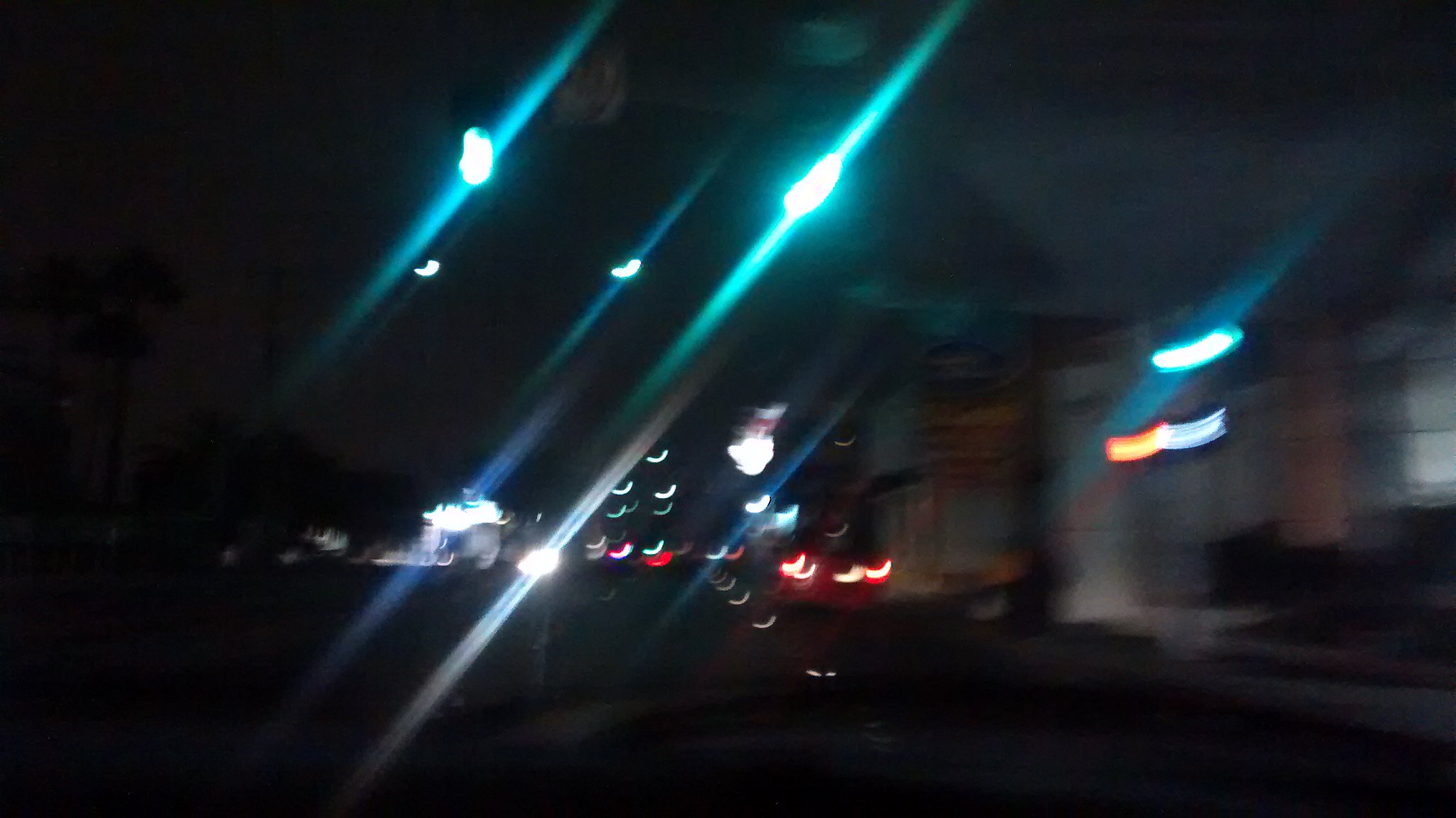This nighttime, color photograph is extremely dark and appears to have been taken in motion, creating a distorted and blurry effect. The scene is likely outdoors, with the upper left showing an incredibly dark sky, perhaps part of a skyline. The centerpiece of the photograph features two very bright lights, possibly from a light pole, casting shimmering reflections across the image. 

The colors in the photograph are predominantly shades of turquoise, white, yellow, orange, and red. Dashes of these colors streak across the scene, implying motion. Additional white lights are noticeable, some trailing down from above and reflecting off the ground or nearby surfaces. These reflections create various bright spots and patches.

On the right side, there appear to be thick white columns, their attachments unclear. There are also blurred shapes that might be building structures, including glass window fronts where some interior lights and black furniture are faintly visible. The bottom right could hint at a street, though the details are obscured by numerous light reflections.

Amidst this chaotic array of colors and lights, there is a cluster of little knobby white objects on descending lines of light, which may be reflections or part of a structure. Additionally, small shapes resembling birds add to the mystery of the image. Near the center left, there's a barely discernible figure with a white collar, standing in the midst of four red crescent moon reflections.